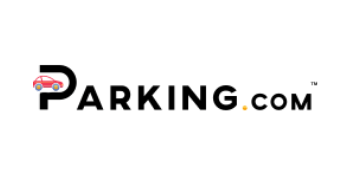The image features the logo for Parking.com. It consists of "Parking.com" in sleek black text, concluded with a small "TM" at the end, indicating that it is a trademark. The background is entirely white, creating a strong visual contrast. The distinctive feature is the letter "P" in “Parking,” which contains a stylized, cartoonish red car with yellow and black wheels, adding a playful and memorable touch to the logo. Additionally, the dot in ".com" is highlighted by being yellow instead of black, contributing further to the logo's vibrant and eye-catching design. The clean, white background underscores the elements of the logo, making it suitable for marketing purposes, whether on their website, in advertisements, or other branding materials. This logo effectively communicates the brand's focus and invites viewers to visit Parking.com for more information.